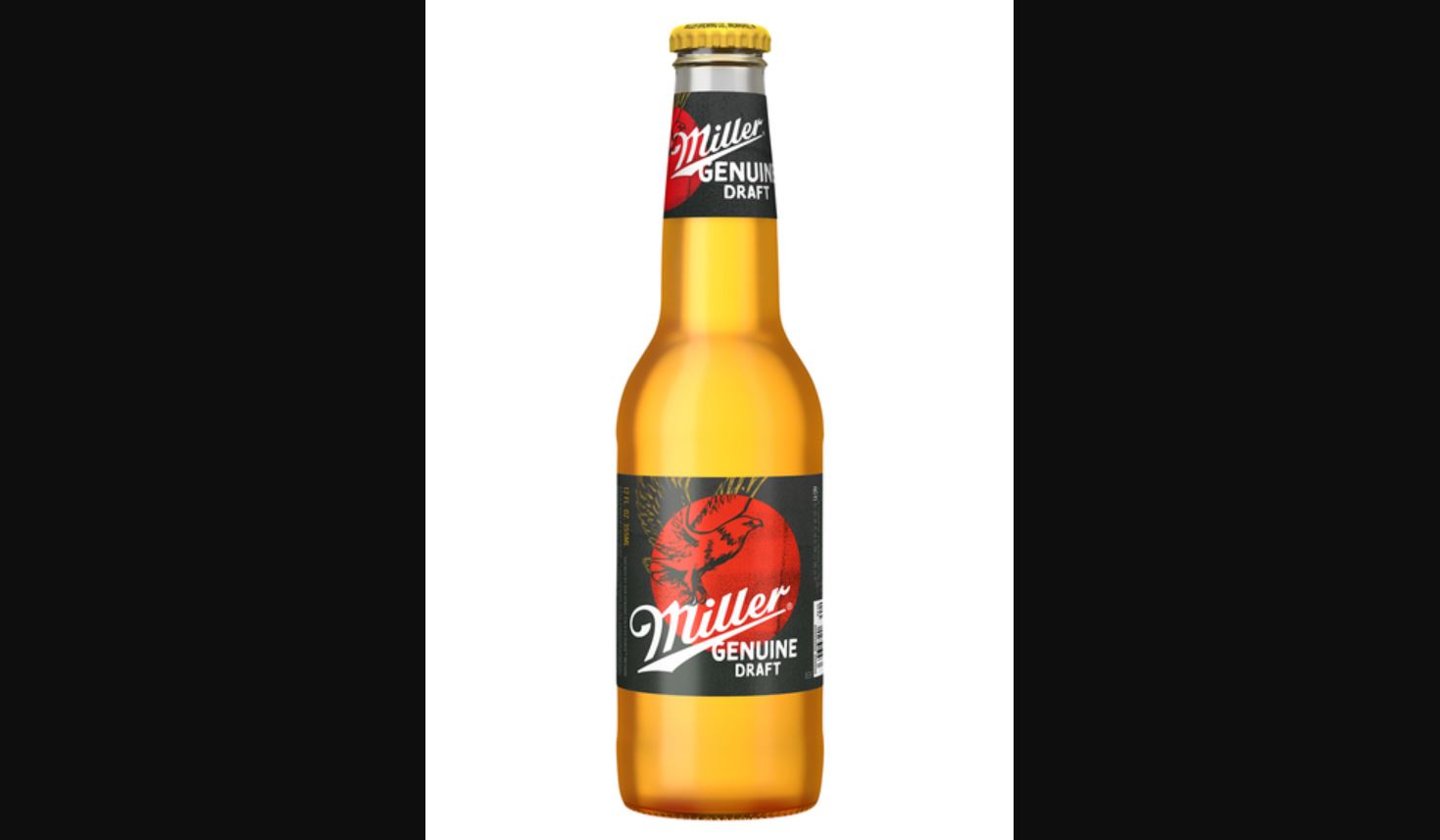The image showcases a digital poster centered on a bottle of Miller Genuine Draft beer, meticulously highlighted against a stark white background with large black borders on both sides. The bottle, golden yellow in color and topped with a yellow cap, stands sealed and full. Prominent on the bottle is a black label, positioned around its midsection, adorned with the text "Miller Genuine Draft." An intricate design features a red circle behind the brand name, within which an eagle, outlined in black and yellow, partially emerges. The neck of the bottle mirrors this design with a smaller label that also reads "Miller Genuine Draft" and features the same red circle and eagle motif. A UPC barcode is located on the right side of the lower label. The rich detail of the bottle's imagery and labels, combined with the striking background, make the poster visually compelling and easy to recognize.